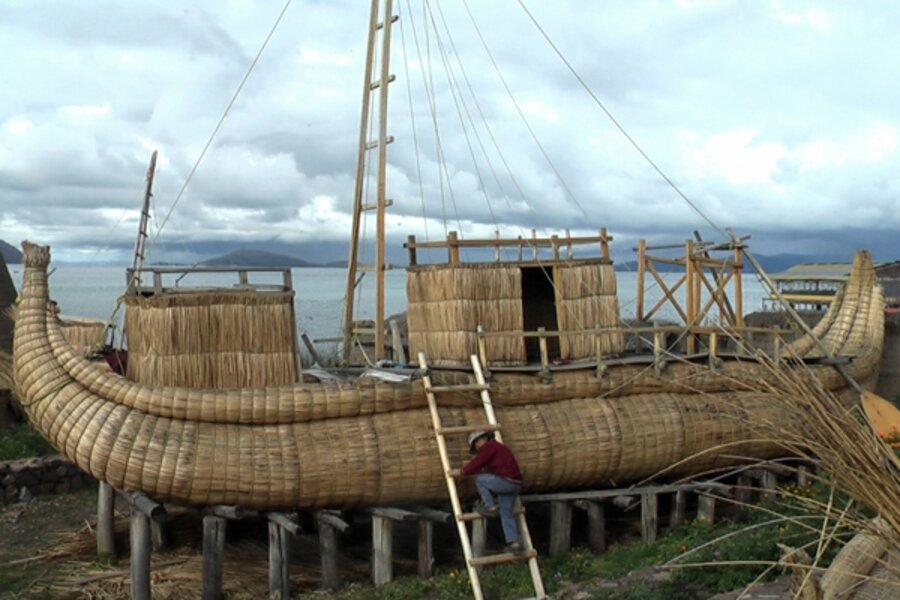The image captures a large, unfinished boat, potentially crafted from thick bamboo or materials resembling straw, resting on wooden pylons and logs. The boat features sloping fronts and backs with small huts on its deck, yet to be fully completed as indicated by the absent sails. Centered in the foreground is a man in blue jeans, a red shirt, and a hat, ascending a homemade wooden ladder towards the boat. The background reveals a body of water dotted with distant islands and hills, all under a heavily clouded sky.